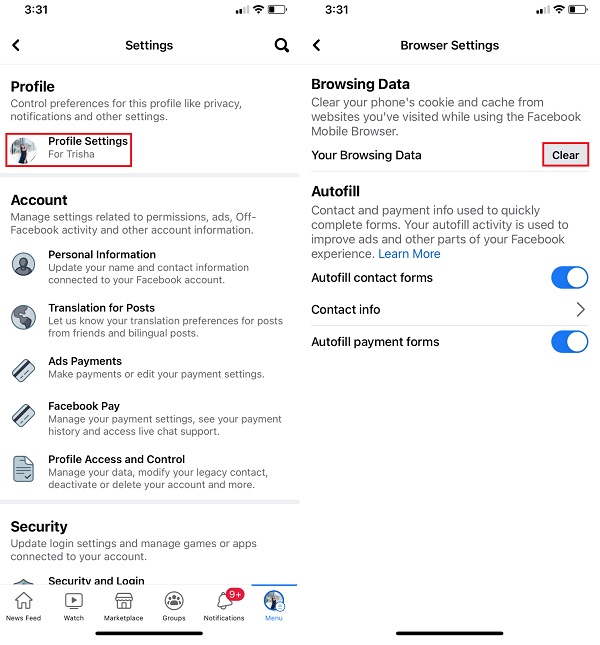The image features two smartphone screenshots placed side by side, each displaying the time "3:31" at the top. On the left screenshot, the main heading reads "Settings," followed by a subheading "Profile." The description underneath indicates that you can control preferences for this profile, such as privacy, notifications, and other settings. A highlighted red box surrounds the section titled "Profile Settings for Tricia."

Below the highlighted section, there are several additional categories listed:

1. **Account:** Manage settings related to permissions, ads, Facebook activity, and other account information.
2. **Personal Information:** Update your name and contact information connected to your Facebook account.
3. **Translation for Posts:** Indicate your translation preferences or performance for posts from friends and bilingual posts.
4. **Add Payments:** Make payments or edit your payment settings.
5. **Facebook Pay:** Manage your payment settings.

Overall, the screenshots capture a detailed view of various customizable settings within a Facebook account, emphasizing the "Profile Settings for Tricia."